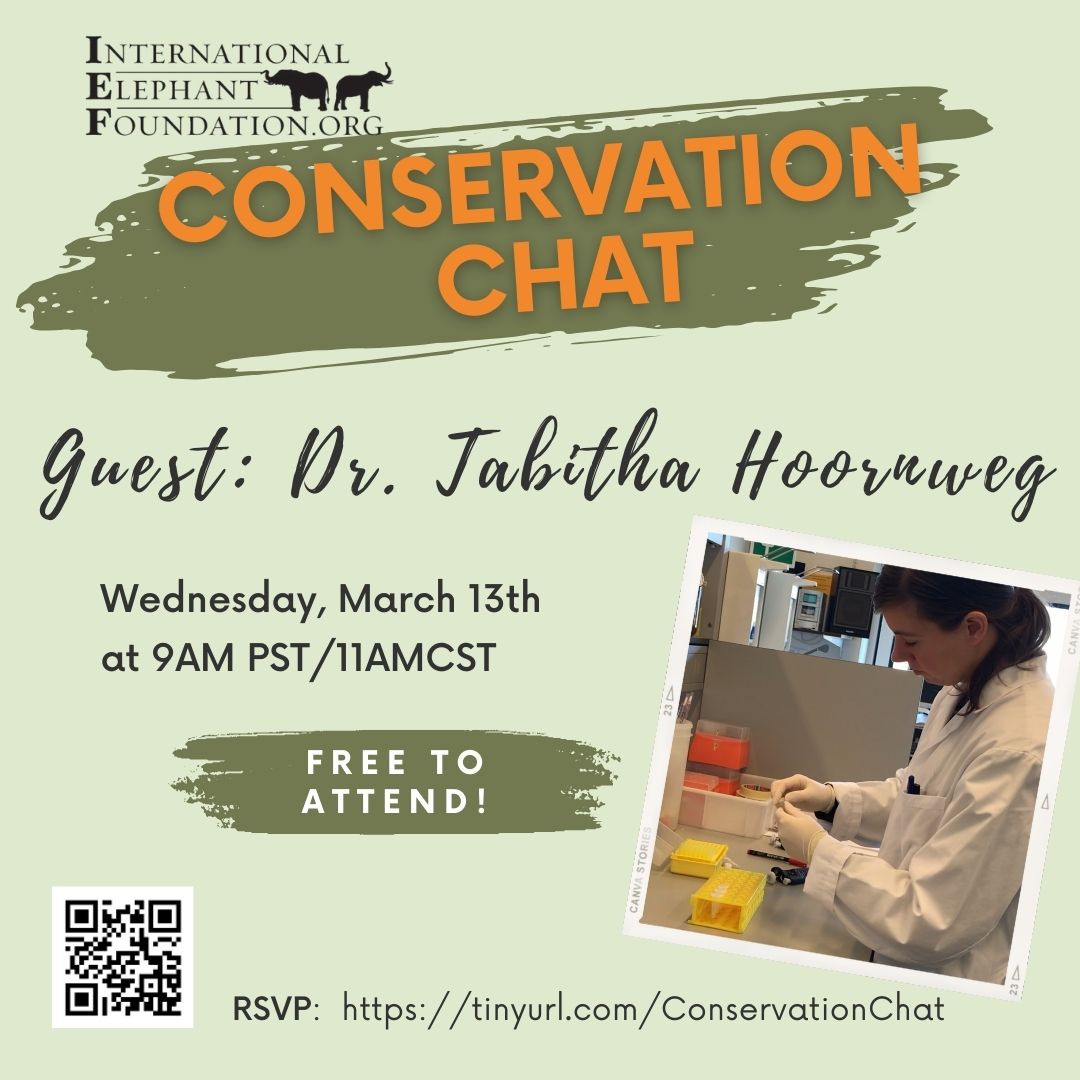This is a detailed invitation for a conservation event hosted by the International Elephant Foundation. The invitation features a white background with a faint light green overlay, giving it a clean and subtle look. In the top left corner, "International Elephant Foundation.org" is prominently displayed, with each word's initial ("I", "E", "F") in bold black accompanied by two small black elephants to denote the organization. 

The main event, titled "Conservation Chat," is highlighted in large orange blocky letters on an olive green backdrop. Below this, the invitation introduces the guest speaker, Dr. Jabitha Hoorweg, and provides the event details: Wednesday, March 13th at 9 a.m. PST / 11 a.m. CST, with a note that it is free to attend. In smaller text, the RSVP link is provided: https://tinyurl.com/conservationchat, accompanied by a QR code on the left for easy scanning.

In the bottom right corner of the flyer, there is a photograph of Dr. Hoorweg. She is seen working in a laboratory, dressed in a white lab coat and rubber gloves, standing over a counter with yellow trays. The background reveals various lab equipment, including a red Sharps container.

Overall, the flyer employs a cohesive green color scheme with splashes of orange and black to emphasize key details, ensuring clarity and visual appeal.